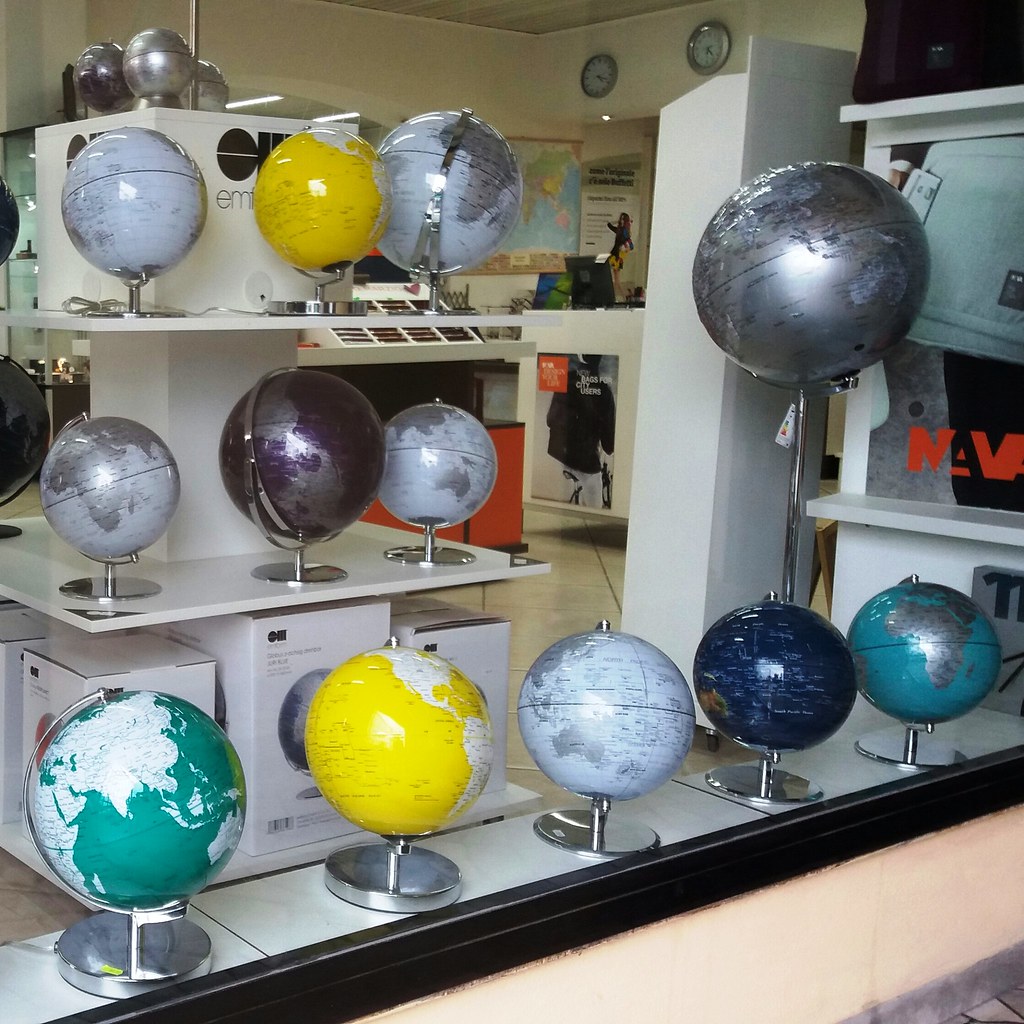The image captures the interior of a modern globe shop, showcasing a diverse and colorful display of globes of various sizes and styles. In the foreground, a bottom shelf features five globes, each with distinct color schemes: one has dark green seas and white landmasses, another has yellow oceans and white lands, and others are colored in light blue, gray, and teal hues, all mounted on sleek silver stands. These globes are arranged meticulously from left to right, prominently displaying their unique designs.

In the background, a two-tiered shelf holds additional globes. On the top row, a white box sits centrally behind a blue globe. The adjacent globes have red seas with white land and light blue seas with dark gray continents. The middle shelf displays smaller yet equally vibrant globes, including a purple one with gray landmasses and another with aqua blue water and silver land. Beneath these, the bottom shelf is also lined with boxed globes, indicating they are new merchandise.

To the right of this elaborate display, a white desk with writing and a picture is visible. A significant column stands out in the center of the room, adding to the layout's symmetry. The shop’s walls feature maps, posters, and a clock, adding to the educational ambiance. Centered above the counter is a notable poster of a man on a bicycle. This meticulous arrangement of globes, combined with the shop's modern design elements, suggests a space dedicated to offering a wide range of globes ideal for educational and decorative purposes.